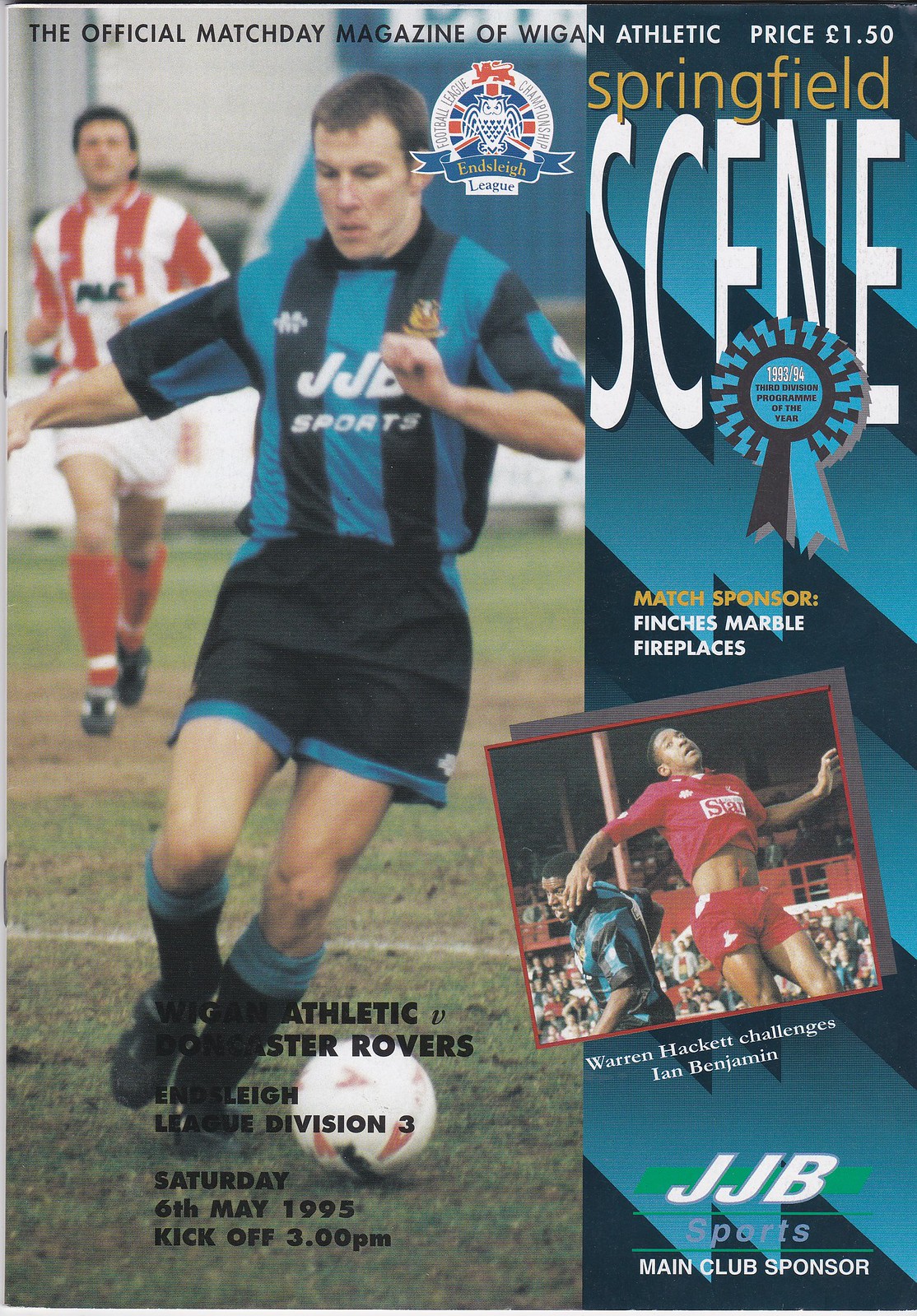The front cover of this rectangular, vintage magazine prominently features the official match day program for Wigan Athletic, an English football club. The title at the top reads "The Official Match Day Magazine of Wigan Athletic," with "Wigan" in black and transitioning to white for "Athletic." Priced at £1.50, the cover is distinctly split into two sides, with the left side dominated by an action photograph of a Caucasian Wigan Athletic player in a blue and black vertically striped jersey, black shorts with blue trim, and knee-high black socks. The player appears to be either chasing or about to kick a soccer ball, with a blurred red and white vertically striped uniformed opposition player from Doncaster Rovers in pursuit behind him.

The right side of the magazine has a blue background with jagged blue and black lightning-bolt patterns. Across this section, there's yellow and white text that reads "Springfield Scene." An additional highlight of the cover includes various advertisements and sponsorships. A small blue ribbon signifies the magazine's accolade as the "1993-94 Third Division Program of the Year." Below this, in yellow, the "Match Sponsor" Finch's Marble Fireplaces is noted, and further down, JJB Sports is acknowledged as the main club sponsor.

Near the bottom left, the publication provides details of the featured match – Wigan Athletic versus Doncaster Rovers, scheduled for Saturday, May 6, 1995, in the Endsleigh League Division 3, with a kickoff at 3:00 p.m. On the right-hand side, an additional square photo depicts two footballers of African descent in mid-action, identified as Warren Hackett and Ian Benjamin, with Hackett in a red and white kit jumping in the air and Benjamin in a blue and black striped shirt behind him.